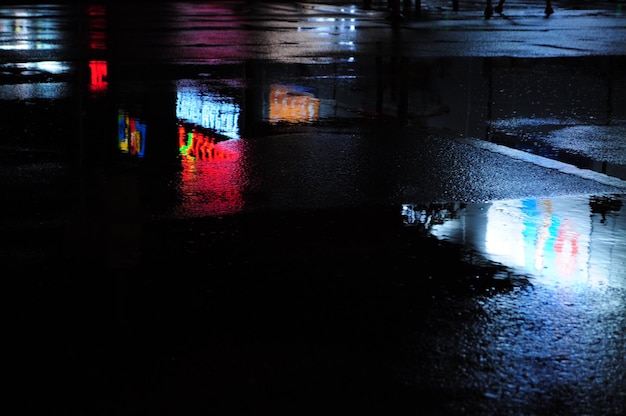The photograph captures a wet asphalt street at night, likely a parking lot, illuminated by the reflections of various neon and lit-up signs in the puddles scattered across the surface. The scene is enriched by the vibrant hues of red, blue, white, yellow, orange, and pinkish purple lights, which create a striking contrast against the dark, rain-soaked ground. Among the notable reflections are a blue and white sign on the right, a prominent neon red sign in the middle, multiple blue, red, and yellow signs to the left, and an orange sign further to the right. The bluish cast of the pavement and the barely discernible feet of distant pedestrians add depth and atmosphere to the night-time setting, enhancing the sense of a bustling yet rainy urban environment.